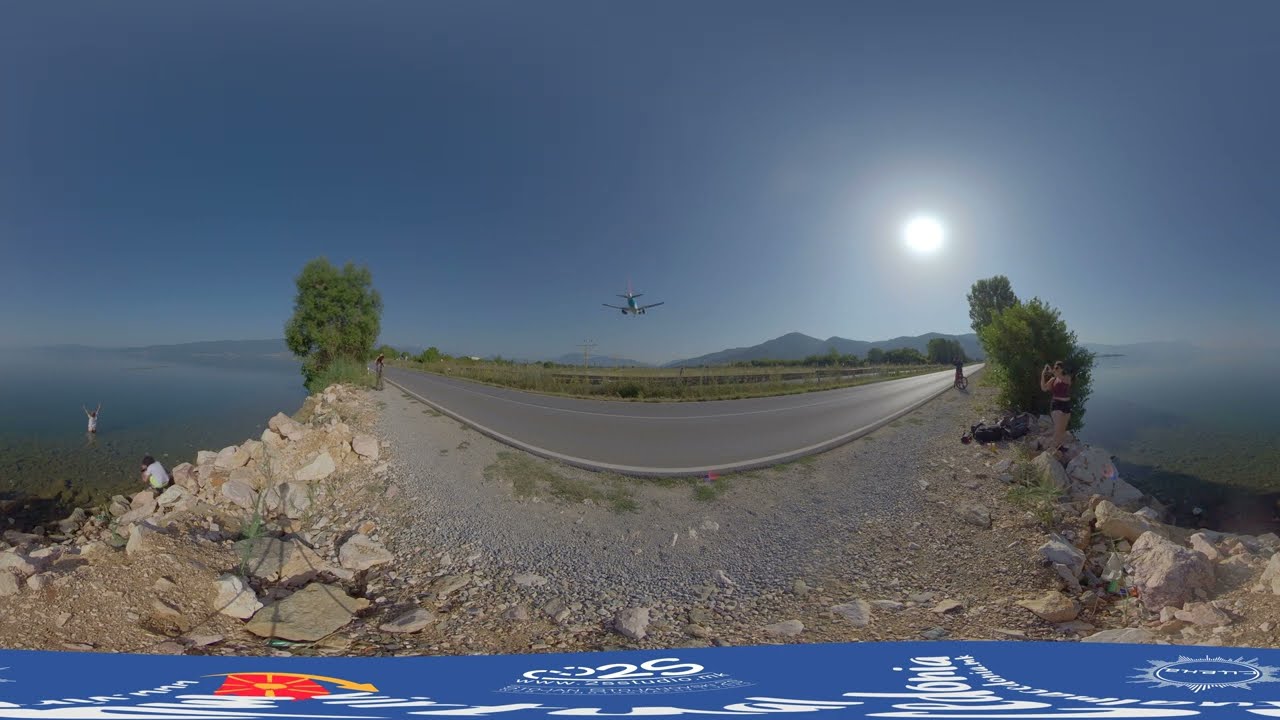This 360-degree panoramic image captures a serene landscape where a white commercial airplane is either landing or taking off from a clear runway. Positioned centrally, the plane faces away from the camera, with the sun shining brightly to its right, illuminating a perfectly clear sky with no clouds. The scene includes a broad road, distinctly curved due to the panoramic effect, flanked by gravel, rocks, and shallow waterways on both sides, which reflect a greenish hue. In the distance, a magnificent mountain range stretches across the horizon.

In the foreground, several people add life to the composition. To the right, a woman in a red tank top and shorts is engrossed in taking a photo. Nearby, another figure stands by the side of the road. On the left, a person stands in the water with their arms raised, while another person, positioned behind them, captures the moment. The bottom of the image features a blue stripe with unreadable text, adding a hint of mystery to this vibrant scene.